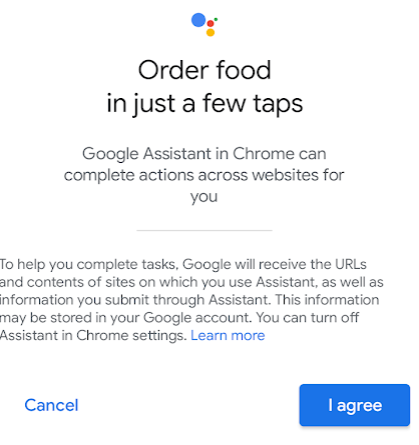Here's the cleaned-up and detailed caption:

---

The image displays a notification from Google Assistant within the Chrome browser. At the top, it features the Google Assistant logo, composed of four multicolored dots: a large blue dot, a small red dot, a medium-sized yellow-orange dot, and a very small green dot, arranged in a distinct pattern. Below the logo in black text, the notification reads, "Order food in just a few taps." Underneath, a description in light gray text states, "Google Assistant in Chrome can complete actions across websites for you."

A faint gray line separates this section from the detailed information below. The lower section elaborates that, "To help you complete tasks, Google will receive the URLs and contents of sites on which you use Assistant, as well as information you submit through Assistant. This information may be stored in your Google account." Further, it mentions that users can disable Assistant in Chrome settings and includes a clickable "Learn more" link in blue text.

At the bottom of the notification, there are two options for the user: "Cancel" in bold blue text and a blue button labeled "I agree" to confirm their consent.

---

This finely detailed caption encapsulates all elements and informational content presented in the image, offering a comprehensive and clear description.